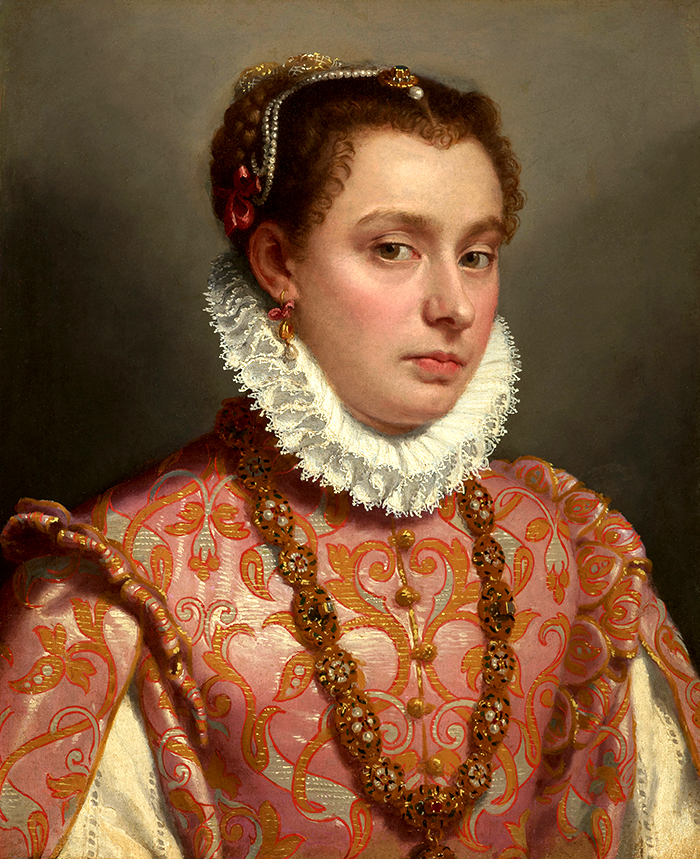The painting is a highly detailed Elizabethan-style portrait of a noblewoman, richly adorned and resplendently attired in lavish garments. She gazes directly at the viewer, exuding an air of discomfort and boredom. Her hair, a reddish-brown color, is styled in loose, short curls but intricately braided and tied back, adorned with gold and green jewelry, pearl beads, and a striking red ribbon on the left side. 

Her high, elaborate collar, indicative of Elizabethan fashion, frames her face, adding an air of regality. Dangling from her ears are elaborate gold earrings with pearls, matching the bejeweled gold and pearl necklace that encircles her neck, reminiscent of ladybugs with its spotted, intricate design. 

The dress itself is opulently crafted from thick, heavy fabric, resplendent in shades of pink and orange with an intricate floral pattern, complemented by regal ruffles and scrolls. The sleeves are uniquely designed, with a split revealing a pale, cream-colored lining beneath. The overall texture and weight of her attire contribute to her evident discomfort, further emphasized by her expression, which clearly conveys a wish to be elsewhere. The background of the painting is a stark, matte black, drawing the viewer's attention solely to the richly detailed figure of the woman.